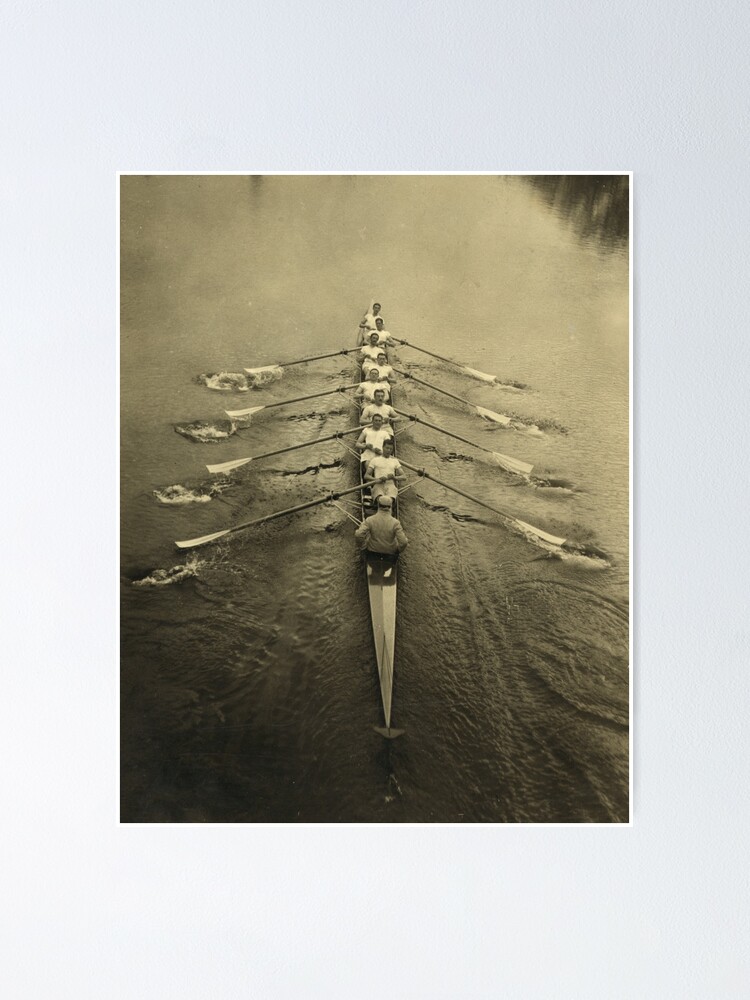In this sepia-toned, vintage image, we observe nine individuals engaged in the sport of crewing, rowing a long, narrow canoe or longboat. The scene is dominated by shades of sepia, lending it an antiquated, almost tea-stained appearance. The boat, which has a long and pointed bow constituting about a third of the image, is seen from a high angle, creating a dynamic composition. Among the nine people, eight rowers are facing the camera, all synchronously lifting their oars out of the water in a coordinated effort, while one individual, presumably the captain, faces them, clad in a darker long-sleeved shirt, distinct from the rowers' white t-shirts. The water in the foreground is dark and agitated by the oars, contrasting with the calm, lighter waters behind them. You can discern the disturbance in the water where each paddle has lifted and dipped. The upper right corner of the image reveals the reflection of a tree, adding an element of natural scenery to the disciplined, athletic endeavor occurring in the boat. The boat appears almost knife-like in its sharpness, enhancing the sense of movement and precision captured in this moment.